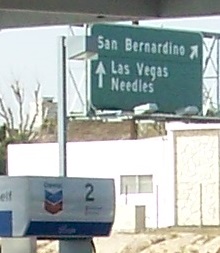In this small, vertically rectangular exterior image, natural lighting illuminates the scene. In the lower left portion of the frame, the top of a gas station pump prominently displays the Chevron logo on a white background, alongside the number "2," indicating pump number 2. The viewer’s perspective is angled upward. In the distance, occupying the upper right portion of the frame, a large green interstate sign mounted on a metal frame directs travelers. The sign reads "San Bernardino" with an arrow pointing to the upper right. Below, another arrow points straight up with the destinations "Las Vegas" and "Needles" indicated.